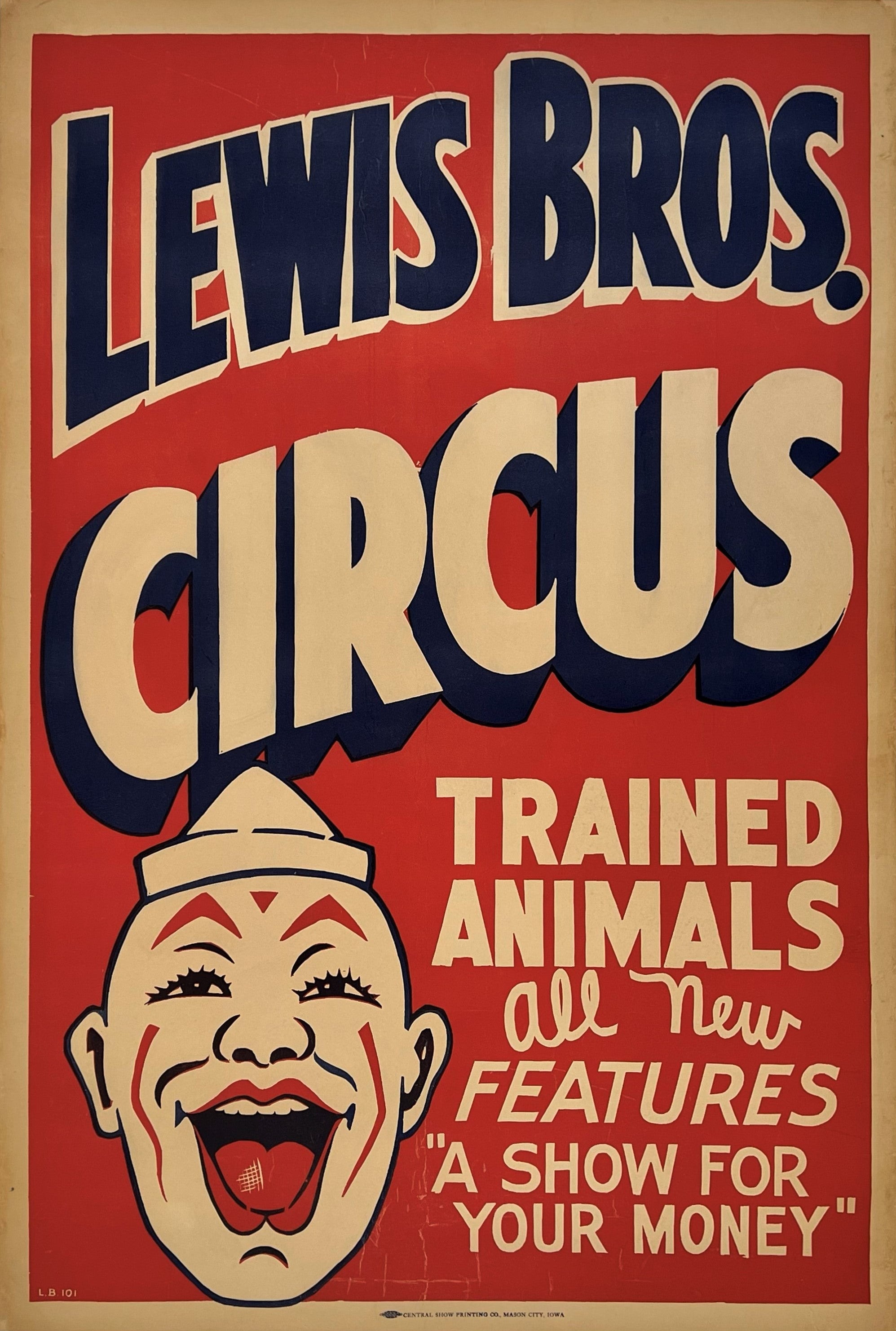This hand-painted poster features an advertisement for the Lewis Bros Circus, prominently displaying the name "Lewis Bros" in bold black letters with a white shadow, followed by the word "CIRCUS" in striking white text with a black shadow. The background is a vivid red, framed by an elegant gold border that encapsulates the entire sign. At the bottom right, additional promotional text in white letters reads: "TRAINED ANIMALS, ALL NEW FEATURES," and in a cursive font, "A SHOW FOR YOUR MONEY." This latter phrase is notably in quotation marks.

To the left of the textual content is a detailed image of a traditional circus clown. This entrancing figure, with tan skin and distinct makeup, features red eyebrows, red cheeks, red lips, and a red tongue – all accentuated by white teeth, which are only visible in the upper jaw. The clown wears a triangular hat resembling a sailboat, detailed with red triangles above the eyes and red lines on the cheeks, adding to the nostalgic feel of the advertisement.

Subtle additional text in gold and black appears at the very bottom of the image, though its small size renders it difficult to decipher. Overall, the poster exudes an old-timey charm, effectively capturing the vibrant and captivating essence of the circus.